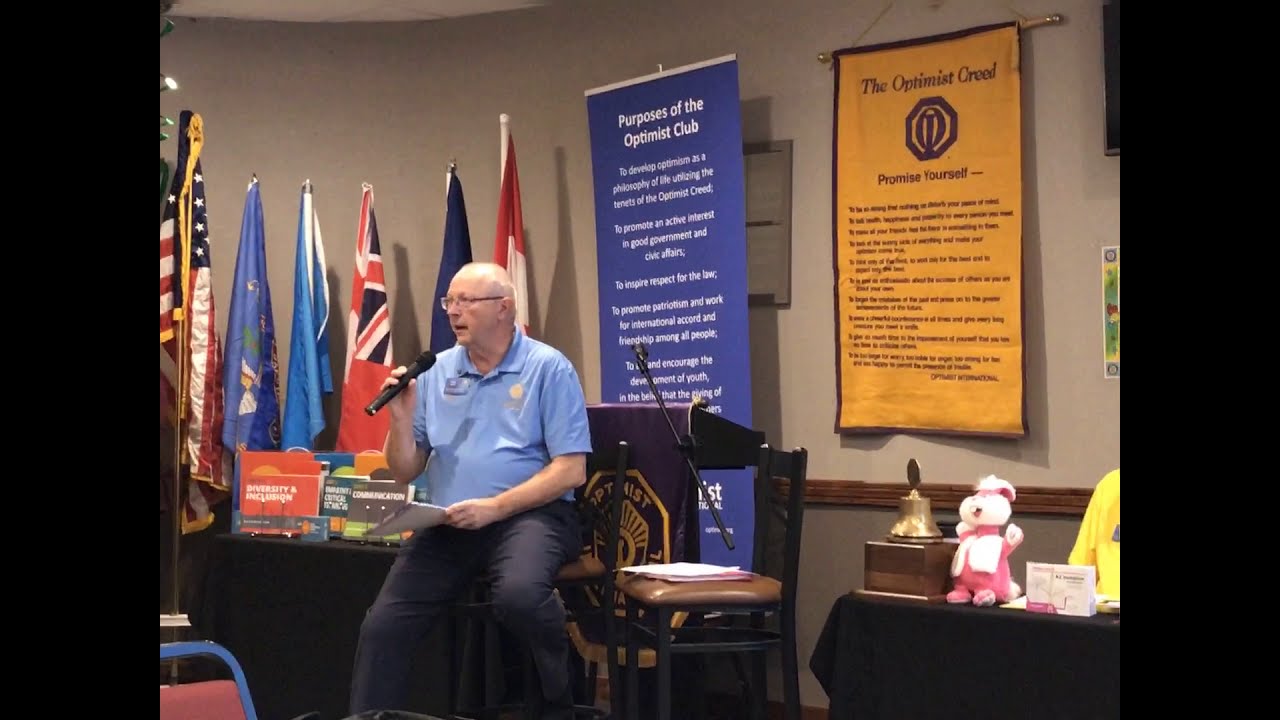In this indoor event setting, an older, balding man with glasses is seated on the edge of a desk. Dressed in gray slacks and a light blue shirt with a badge on his left breast pocket, he holds a black-framed microphone in his right hand and a booklet or cheat sheet in his left. The chair he occupies features a brown leather seat with a black backrest and legs. Behind him, various flags, including the American flag and what appears to be the British flag, hang on white poles with silver tops. These flags are partially obscured and range in colors from blue and green to yellow, red, and white. The wall in the background is tan on top, transitioning to gray below, separated by a brown ledge. A prominent yellow banner with black trim reads "The Optimist Creed," while a blue banner positioned on a stand announces "Purposes of the Optimist Club." In front of the man, a table draped in a black tablecloth holds a pink and white stuffed bunny, a gold bell on a brown box, and nearby, a woman in a yellow shirt is seated. The setting suggests a formal or semi-formal gathering, emphasizing the themes of optimism and purpose.